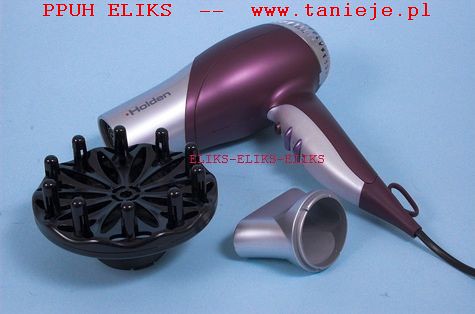The photo features a purple hair dryer with a silver tip, a silver rounded back, and a silver grip area with three buttons. The main body of the dryer is a mix of dark and light purple, and it is shown lying on a light blue background. The back vent is light purple, and a black power cord is attached to the dryer. Next to it, there's a black diffuser attachment with short, plastic spokes, as well as a silver nozzle attachment. At the top of the image, in red capital letters, is the text: "PPUH ELIKS -- www.tanieje.pl". Similar red text in the middle of the image reads: "ELIKS-ELIKS-ELIKS".